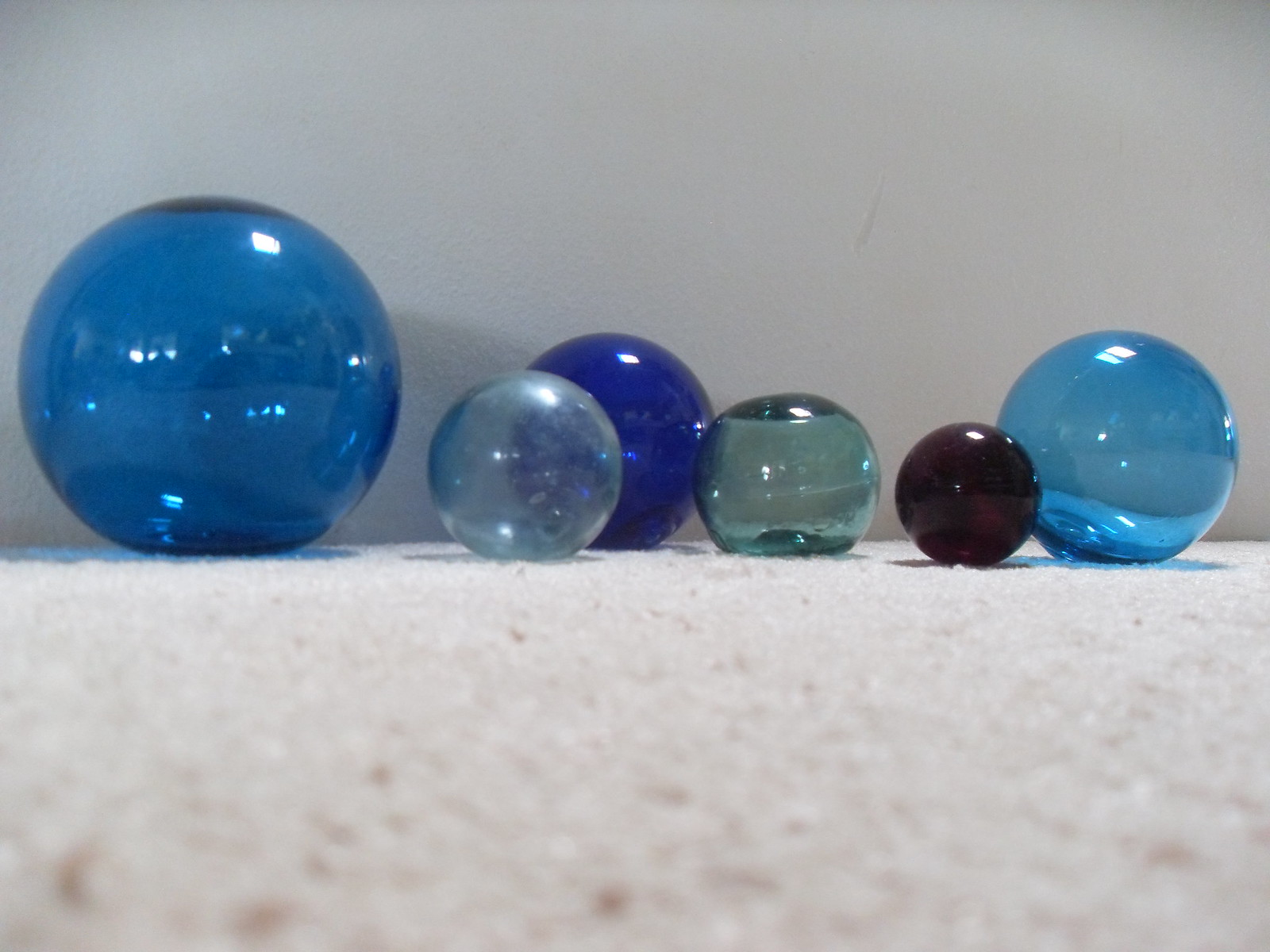This image features six translucent glass balls of various sizes and colors, arranged on a surface that appears to be white carpet but could also be interpreted as a slightly dirty ground. The background is a light gray to off-white wall. On the left, there is a spherical ball of medium blue color with flecks of light reflecting off its surface, approximately three and a half to four inches tall. Next to it, there's a smaller, almost clear blue ball, around one and a half to two inches in height. Moving right, a slightly taller ball of vivid royal blue hue, followed by a crystal-clear ball with a hint of greenish shade, reminiscent of a glass bottle. Further along, there is a completely opaque dark gray ball. Finally, on the far right side, is a larger dark blue ball with little square light flecks along the top, standing about three inches tall. The differing descriptions converge to highlight the variety in size and the unique, striking colors of the glass balls.